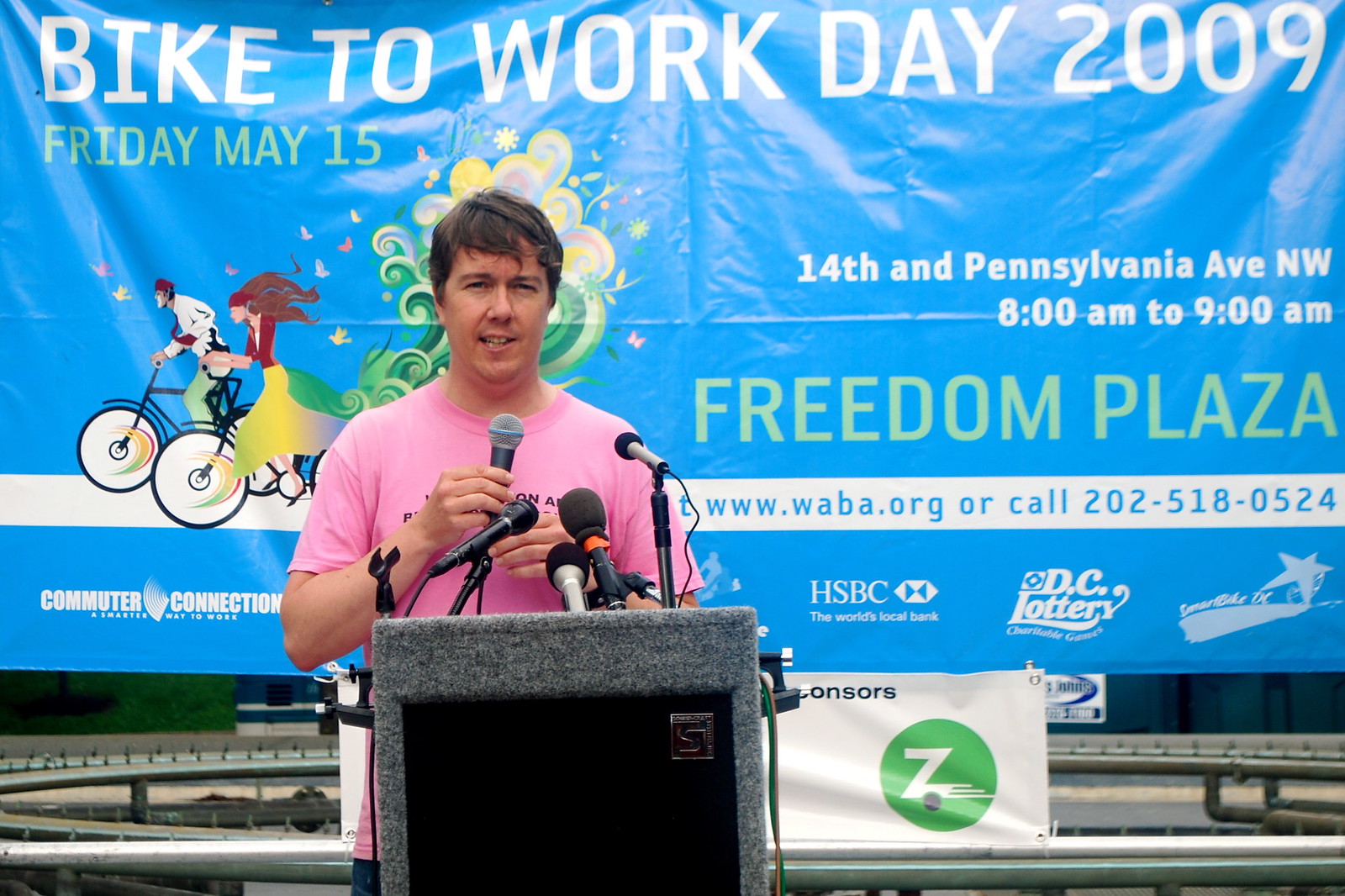In this outdoor photograph, a man with short dark hair and clean-shaven face stands under natural lighting at a black podium with a gray border, surrounded by several microphones, including one he holds in his hand. He is mid-sentence, likely encouraging participation in "Bike to Work Day 2009," as indicated by the large, bright blue banner behind him. The banner prominently features white and yellow text detailing the event date, Friday, May 15th, and location at 14th and Pennsylvania Avenue, NW from 8 a.m. to 9 a.m., as well as the venue, Freedom Plaza. Additional information on the banner includes the website www.wabba.org and the contact number 202-518-0524. Decorative elements on the banner include cartoonish images of two cyclists. The man is dressed in a short-sleeved pink T-shirt, focused on delivering his speech.